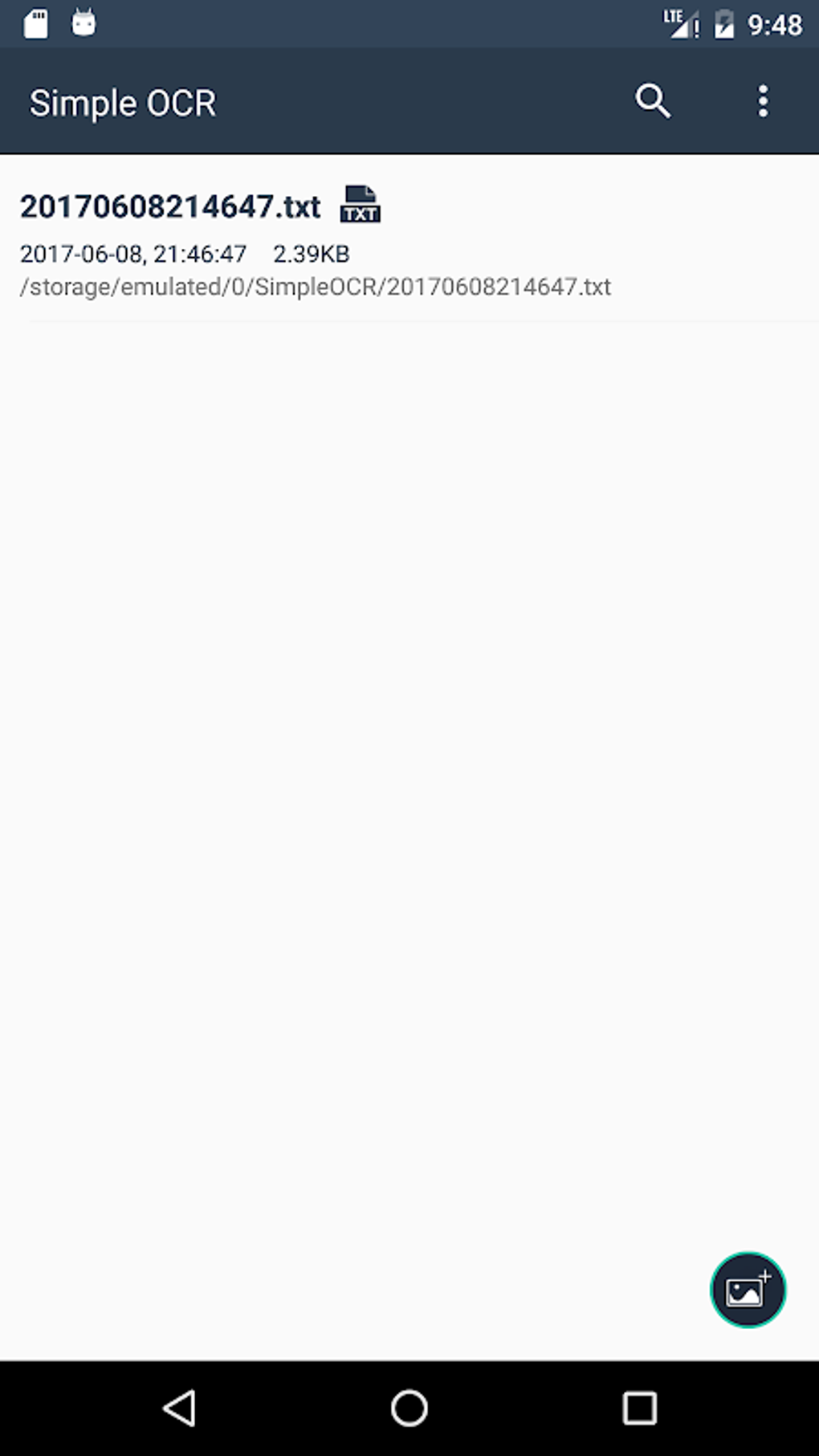The image showcases a very plain and minimalistic website interface displayed on a smartphone. At the top, the site prominently features the title "Simple OCR" in a dark box. The status bar of the phone shows a time of 9:48, a battery life at around 50%, and an LTE connection.

Below the title, a string of numbers is displayed: "201-706-082-14647." This is followed by the label "Text" accompanied by a small text image. Further details provided include "2017-06-0821...46...47" and the file size "2.39 KB." There is a mention of a directory path: "storage/emulated/0/simple OCR/201-706-082-14647 text."

At the bottom of the website, a dark round circle outlined in light blue is present. Inside this circle is a box featuring white hills with a small plus sign in its upper right corner, potentially indicating an upload or add button. The image also includes standard smartphone interface icons at the bottom.